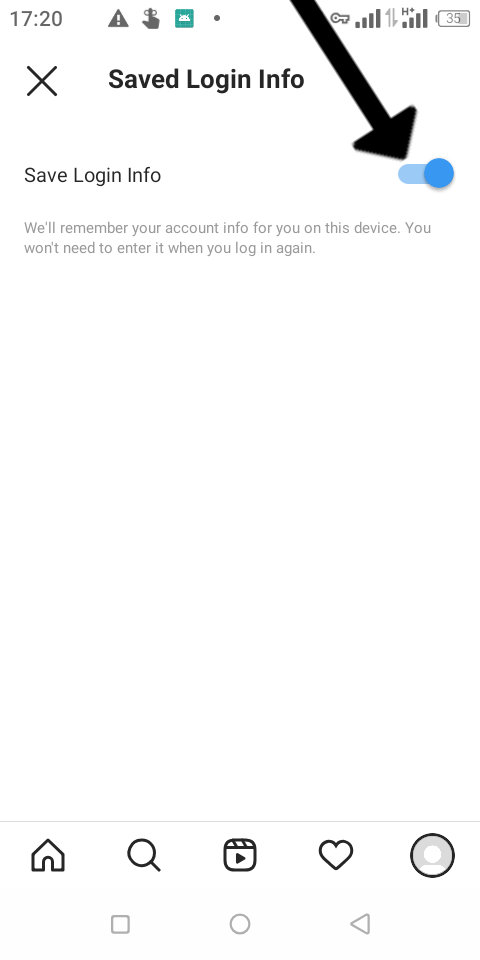The image consists of a vertical screenshot of a mobile application interface, displayed on a white background. 

At the very top, the status bar shows the time "17:20" in the left corner, accompanied by various app icons. On the right side, the battery icon indicates a 35% charge and four bars of signal strength.

Below the status bar, a centered bold text heading reads “Save login info,” followed by a smaller, lighter text repeating the same phrase. To the left of the bold heading, there's an 'X' icon.

Directly beneath this section, a toggle switch is visibly turned on, exhibiting a blue color. This switch is likely used to enable the saving of login information on the device. Accompanying text states, "Remember your account info for you on this device," and includes additional details over two lines.

At the bottom of the screen, common navigation icons such as 'Home' and 'Videos' are visible, suggesting this is a typical smartphone interface. A prominent black arrow, apparently drawn manually, points towards the blue toggle switch, emphasizing its significance in the context of the image.